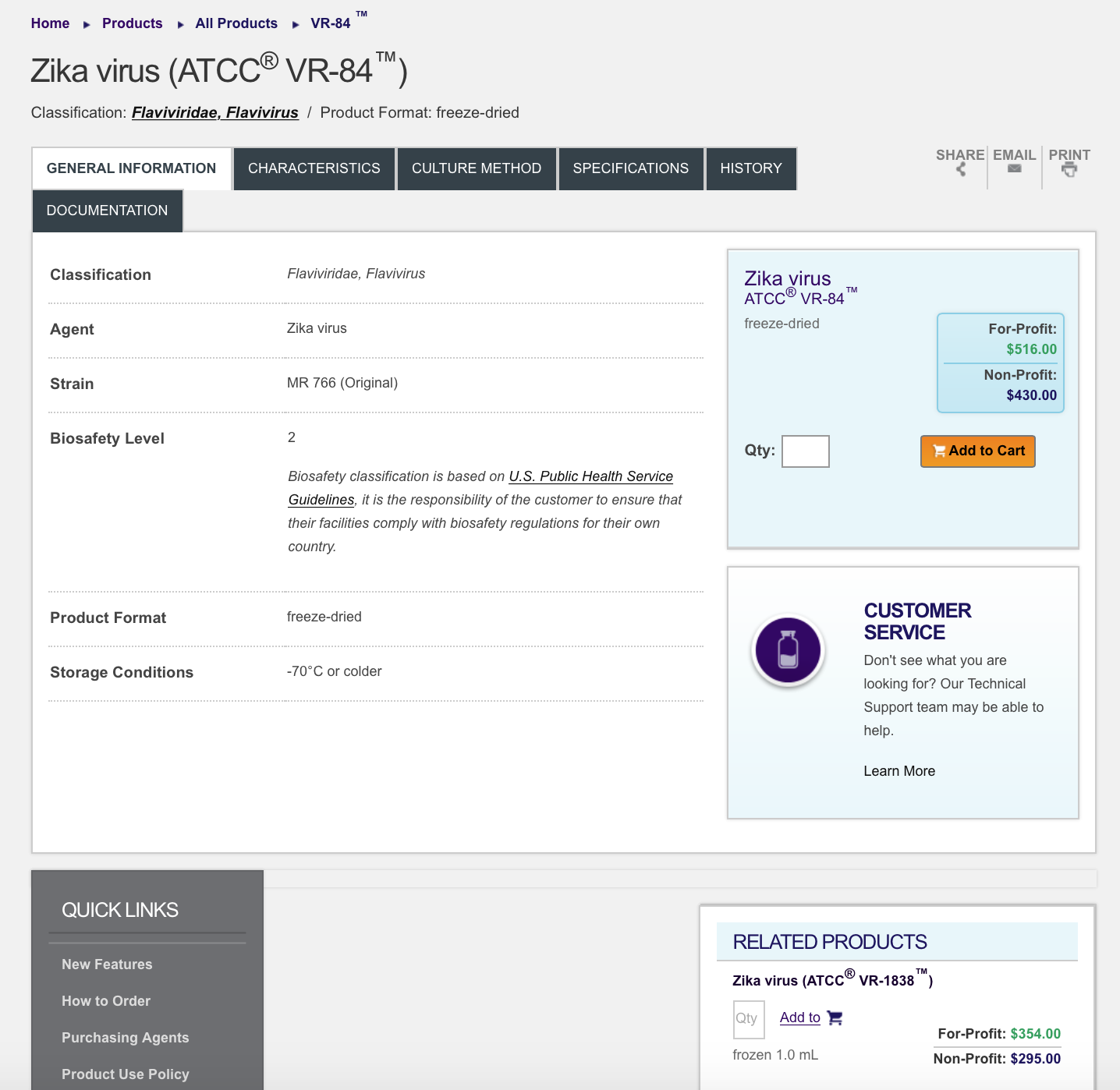This is a detailed screenshot of a website with a gray background. In the upper left corner, blue text labels navigational links: "Home" with a right-pointing arrow, followed by "Products," "All Products," and finally "VR-84TM." 

Directly below, in black font, the text reads: "Zika virus (ATCC VR-84TM)." Further down, the description continues with "Classification: Flavivirus, Flaviviridae. Product Format: Freeze-dried."

Immediately underneath, there are several navigation tabs. The first tab, labeled "General Information," is white and has been selected. The adjacent tabs, shaded in gray, are labeled "Characteristics," "Culture Method," "Specification," "History," and "Documentation." Towards the right of these tabs, there are icons for sharing via email and printing.

Beneath this section, towards the top, a white square contains more detailed classification information: "Flavivirus, Flaviviridae, Agent: Zika virus, Strain: MR-766, Original, Biosafety Level 2." An additional note clarifies: "Biosafety classification is based on the U.S. Public Health Service guidelines."